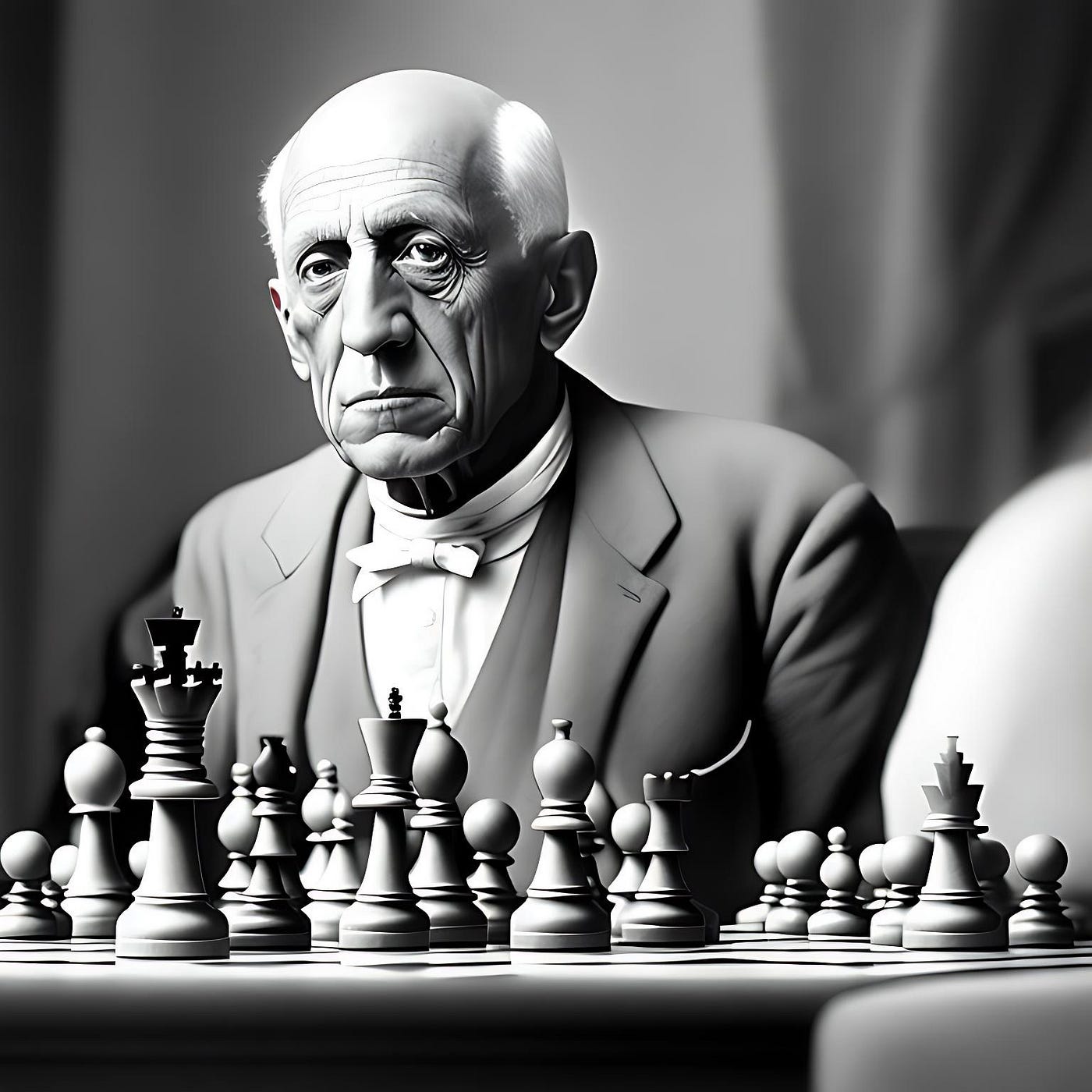This is a detailed black and white drawing, possibly AI-generated or hand-drawn, of an elderly man seated at a chessboard. The artwork features high contrast, highlighting the expressive, wrinkled face of the man, who is bald with some grey hair on the sides. He is dressed in a grey suit, a white shirt, and a bow tie, which suggests a formal or special occasion, possibly even a master's chess tournament. The man, who looks weary or contemplative, is not focused on the chess pieces in front of him but is instead staring outward, giving an impression of deep thought or sadness.

The chess set in front of him is basic, with a distinct king piece standing out, possibly symbolizing the man's own isolation or status. The background is out of focus, hinting at a blurred curtain or stage setting, adding to the somber and introspective atmosphere of the scene. To his right, there is a white shape, perhaps a chair, indicating the presence of another person or just adding to the complexity of the image's composition.